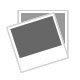This image appears to be a detailed, multi-part advertisement focusing on retro automotive components and vehicles. The main, dominant image at the top features a vintage motorcycle taillight, identifiable by its aluminum-colored cylindrical body with a rounded end and two black wires emerging from it, which later split into red and black wires. The taillight has "STOP" prominently displayed across its face. Reflected beneath it, the taillight is shown on a glossy black table, adding a sharp, mirrored effect. In the upper-left corner of this section, there's a red inscription which seems to say "MOFO Motorcycle".

Beneath this primary image, the visual content is divided into two smaller photographs. On the bottom left, there is an old-fashioned black pickup truck, standing out with its red wheels and thin tires, parked in front of a garage-like setting. It has a distinct tall, boxy cab and a very short bed, characteristic of vintage designs. To the right of this truck image, another photograph presents the rear view of a classic car, likely from the 1950s. This car is gray with a spare tire mounted on its back, the tire rim painted yellow and secured with a chrome attacher. The striking detail of the chrome wheel well and the overall pristine condition of these vehicles suggest that they might have been restored, preserving their antique charm.

Collectively, this triptych forms a compelling advertisement that showcases the aesthetic beauty and intricate detailing of vintage automotive parts and vehicles.